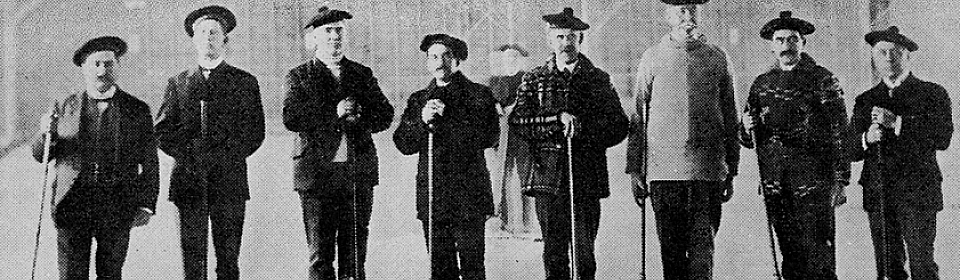This is a horizontal black-and-white photograph, likely from olden times, featuring a group of eight men standing in a line, with a blurred figure of a woman in a long dress and scarf in the background. The men, who vary in height, are all wearing similar round hats, each topped with a small pom-pom, and dark slacks. Many sport facial hair; four or five have mustaches, while three are clean-shaven. Most are dressed in suit jackets, though one man stands out in a lighter-colored jacket. They all hold slender cane-like poles, some with one hand and others with both. The backdrop, a fuzzy but contrasting mix of white and dark gray areas, suggests a wooded area or possibly a trestle structure. Their serious expressions and uniform stance give the impression of a formal gathering, captured sharply against the indistinct background.